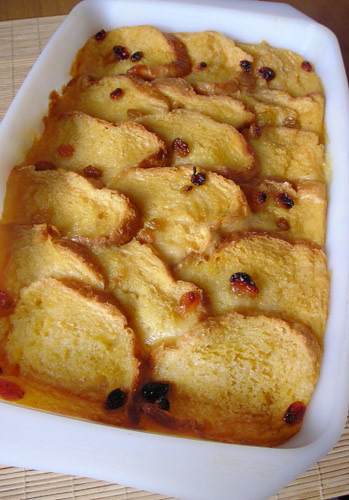A rectangular white ceramic dish, approximately 9 by 14 inches, is filled with golden yellow bread pudding made from roughly 15 slices of white bread dipped in egg batter and baked. The bread, which retains its crust, is arranged in neatly overlapping layers, interspersed with raisins and specks of red fruit, likely cranberries, adding pops of color. The dish's surface appears soft and gooey with a slight toasted texture. The pan is slightly askew, angled towards the left of the image. It rests atop a wicker table, or possibly a bamboo mat, with a ceramic-tiled wall providing a muted backdrop. There are subtle shadows cast on the top left portion of the scene, adding a touch of depth to the otherwise homely and inviting setting.